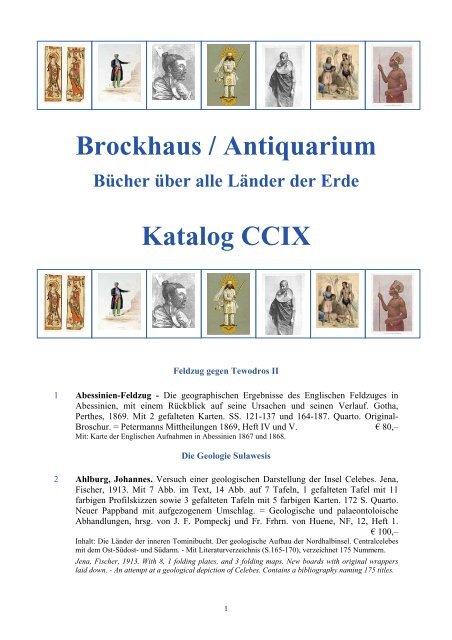The image appears to be a detailed poster or page from a catalog for the Brockhaus Antiquarium, written in what seems to be German. The title "Brockhaus Antiquarium Butcher über alle Lander der Erde Catalog CCIX" is prominently displayed in light blue letters against a white background. The layout includes two identical rows of images, depicting a mix of portraits and scenes that might be renowned historical drawings or illustrations of significant figures. The first image shows two individuals staring at each other, followed by a person pointing to the right in the second image. The third and fifth images are black and white portraits of men, while the fourth image remains unclear. The sixth image features two individuals standing together, and the seventh is a colored portrait of someone looking to the left. Beneath the rows of images, smaller text, too small and foreign to be easily legible, likely provides additional information about the catalog's contents and the artists featured within. The design and formatting suggest that this might be an auction catalog or an exhibit guide, intended to showcase and possibly sell or discuss historical artworks and artifacts.